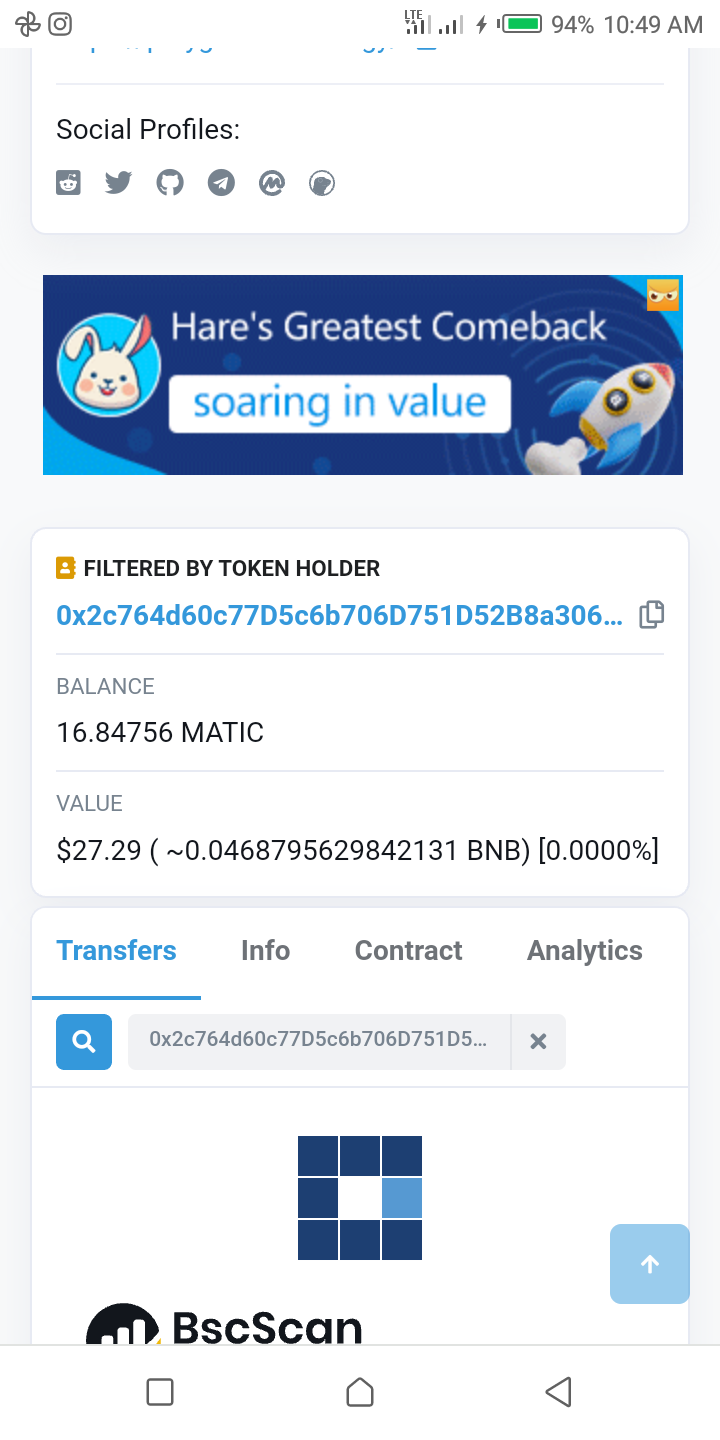This vertically-oriented image, likely captured on a smartphone, features a gray border along the sides while the top and bottom blend into a white computer background. At the top-left corner, small social media icons are visible, while the top-right corner displays the device's signal strength, a battery charge at 94%, and the time 10:49 a.m. 

Beneath this, a section titled "Social Profiles" is accompanied by various popular social media icons. Directly under this section, a blue background hosts the text "Hair is the greatest comeback, soaring in volume" next to an illustration featuring a rocket and a rabbit's face. 

Following this, a white box contains a black text block with an orange icon illustrating a white person figure alongside the text "Filtered By Token Holder" in blue, detailing a long number. This area also displays essential details such as balance and value. Below that, the word "Transfers" is highlighted in blue, accompanied by clickable options for "Info," "Contract," and "Analytics."

Towards the bottom, the interface includes a search bar with an 'X' for closing, followed by a grid layout with squares in navy, lighter blue, and white. The partially visible bottom section ends with the text "BSC Scan" next to a small icon, alongside buttons for navigation: a blue arrow pointing up, a home button, and a left-pointing arrow.